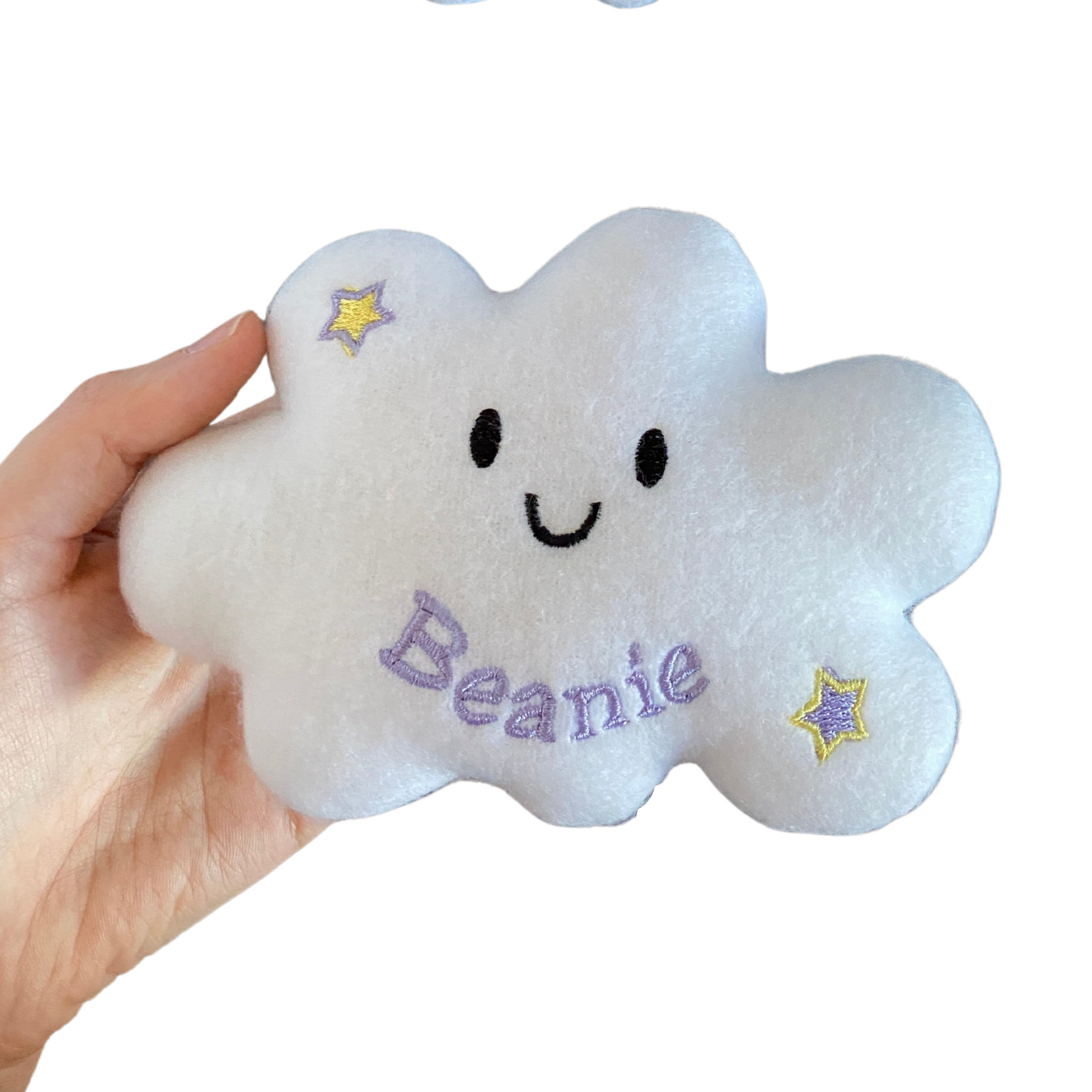The image depicts a left hand holding a soft, cloud-shaped toy with a simple smiley face, characterized by two black oval eyes and a curved smile. The toy has two stars adorning its corners: one in the top left corner featuring a purple border with a yellow center, and a mirrored star in the bottom right corner with a matching purple border and yellow center. The word "BEANIE" is embroidered in purple at the bottom of the toy. The background is pure white, enhancing the prominence of the plushie and the hand holding it.